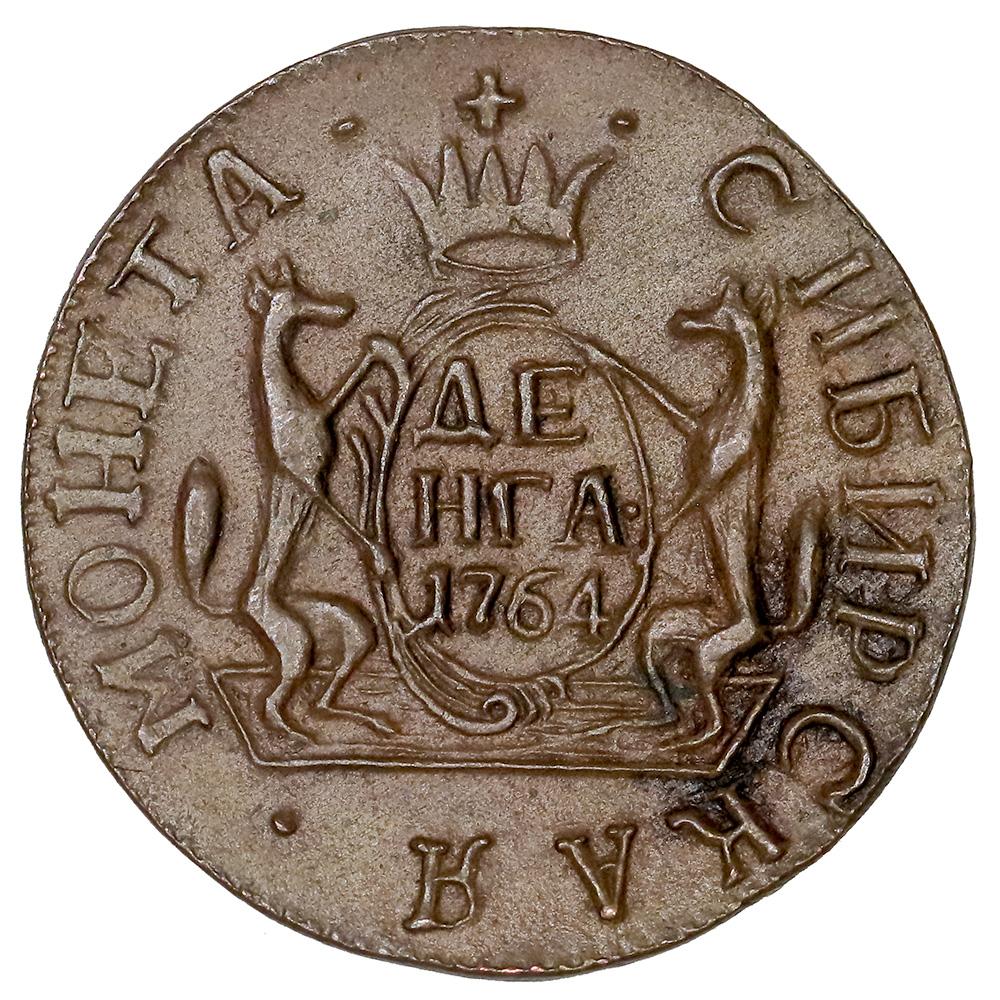This is a very detailed image of a historical bronze coin, displayed against a stark white background without any borders or text. The coin is predominantly round, though it has slight irregularities along its edge, notably on the upper right section where it dips inward slightly, indicative of hand-forging. The surface of the coin is primarily a grayish-brown color.

At the center of the coin, intricate engravings feature two animals, which appear to be kangaroos or possibly foxes, facing each other. Between them, they hold an egg-like shape above which a crown is engraved. Surrounding this central motif are characters that look like they belong to the Cyrillic alphabet, suggesting the coin originates from Russia or a country using a Cyrillic script. These characters include configurations resembling an upside-down 'V' with a line at the bottom, an 'E,' 'H,' an 'A,' and '1764'—likely the date of the coin.

Engraved along the left side of the coin's curve is the word "MOHETA" in capital letters. On the upper right side descending downwards are symbols that include 'C,' a backwards 'N,' a character that looks like a mix between a number '5' and a 'B,' another backwards 'N,' 'P,' then along the bottom, 'C-K-A' followed by one that appears as a backwards 'R'. These letters and symbols further hint at a Cyrillic origin.

Overall, the coin is a testament to the intricate artistry and craftsmanship of the time, enriched with historical significance from the year 1764.